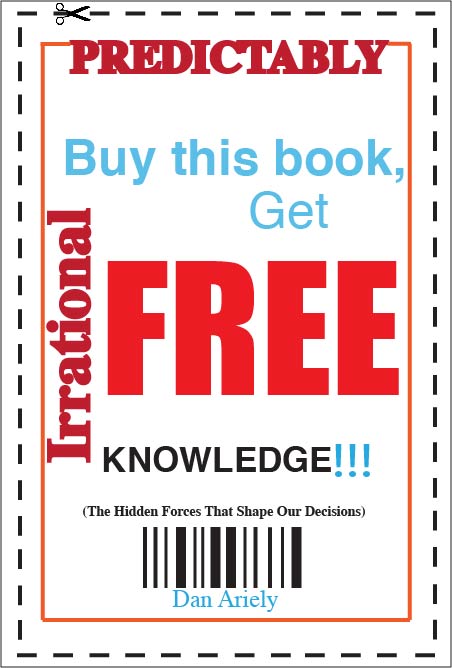The image displays a high-clarity coupon ad on a white background. It features a rectangular design bordered by a dashed cutting line with a scissors icon in the upper left corner. The main text is centrally presented within an orange square line. At the top, the word "PREDICTABILITY" appears in dark red, all capital letters. Beneath it, in light blue text, is the phrase "BUY THIS BOOK" followed by "GET" in the same blue. The word "FREE" is prominently displayed in bold red in the center, and the word "KNOWLEDGE!!!" is at the bottom in black letters with three blue exclamation points. The left side of the coupon has the word "IRRATIONAL" vertically centered in red text. Below the main body of text, a barcode is present, with the name "Dan Ariely" in teal right underneath it. The overall design is colorful, mixing hues of red, light blue, and black, with a white background making the details stand out sharply.